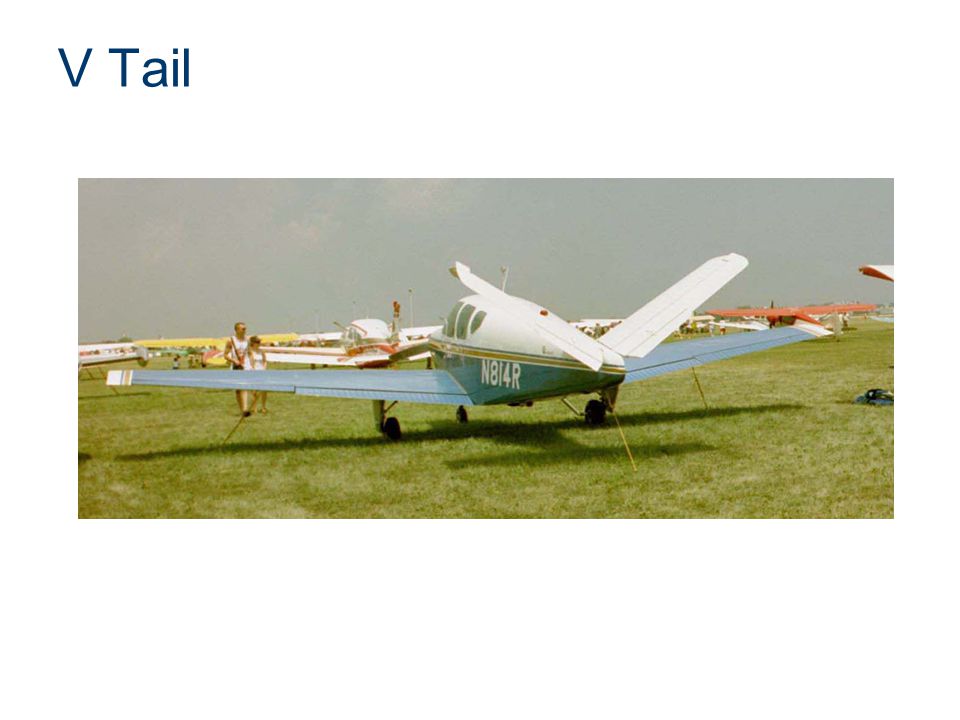In this vintage photograph from the 1980s, the focal point is an old-style small passenger airplane, likely holding around two to ten people. The aircraft, painted in a pristine white with a sky blue lower half, is adorned with a yellow and green stripe down the center and marked with the identifier "N814R" on the side. The top of the plane is marked with red where the wings connect, and the wingtips also feature red stripes. The setting appears to be an outdoor air show at a small airport, with a grassy field extending across the foreground, lush and green. The sky above is notably overcast, with thick gray clouds dominating the scene.

Other small aircraft, including Piper Cubs, Cessnas, and single-engine planes, are visible in the background. They are meticulously tied down at the wings, nose, and tail, potentially as a precaution against high winds. A man and a woman are seen strolling across the grass, likely appreciating the display of aircraft. The central plane is positioned directly in the middle of the photograph, surrounded by this serene yet possibly bustling airshow environment. The textural details of the vibrant red, pink, orange, and yellow hues, along with the diverse aircraft, enrich the nostalgic atmosphere of this snapshot.